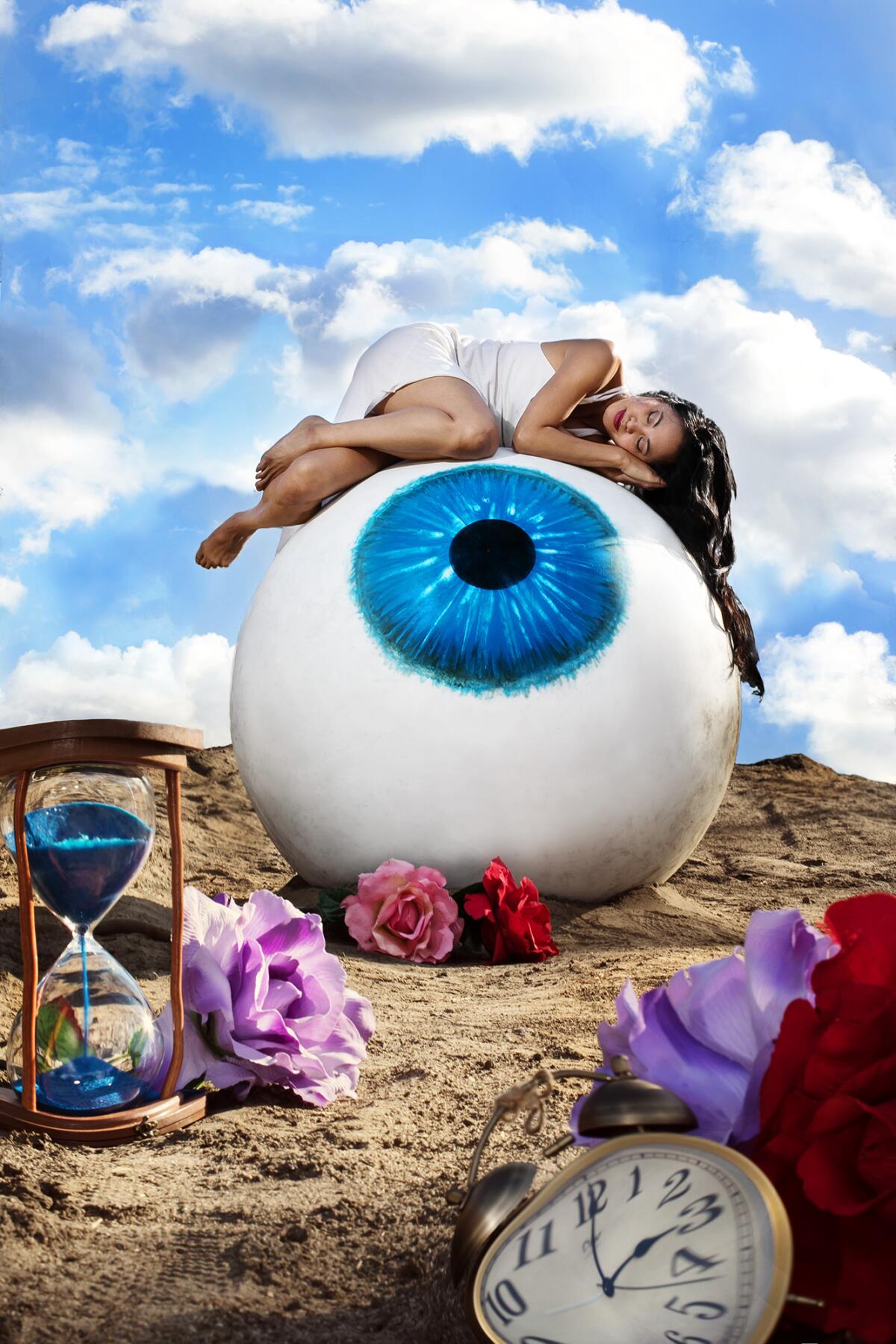This visually captivating artwork, reminiscent of Salvador Dali's avant-garde style, features a hyper-realistic, life-sized diorama set on a serene beach under a sunny sky. The background is a deep blue accented with occasionally scattered, fluffy white clouds that are brilliantly illuminated by natural sunlight. In the center of the scene stands a large, lifelike eyeball with a vivid blue iris, seemingly drawn onto a massive concrete sphere resting on a bed of dry, brown sand. Reclined atop this eyeball is a young woman sporting a short, white dress that leaves her legs and arms exposed. Her long, dark brown hair cascades elegantly down one side of the eyeball as she sleeps, her hands tucked under her head as makeshift pillows.

Encircling the base of the eyeball and embedded in the sand are vibrant flowers, including two red carnations, a pink carnation, and a purple carnation, adding pops of color to the subdued palette. In the foreground to the left, an intricately detailed hourglass with blue sand is enclosed in a wooden frame, the sand steadily trickling down. Adjacent to this, on the lower right, is a classic old-fashioned alarm clock, slightly warped and with its hands pointed to 3 o’clock, creating a surreal juxtaposition with the natural environment. The numbers and hands of the alarm clock are visible, though the clock itself appears to be melting.